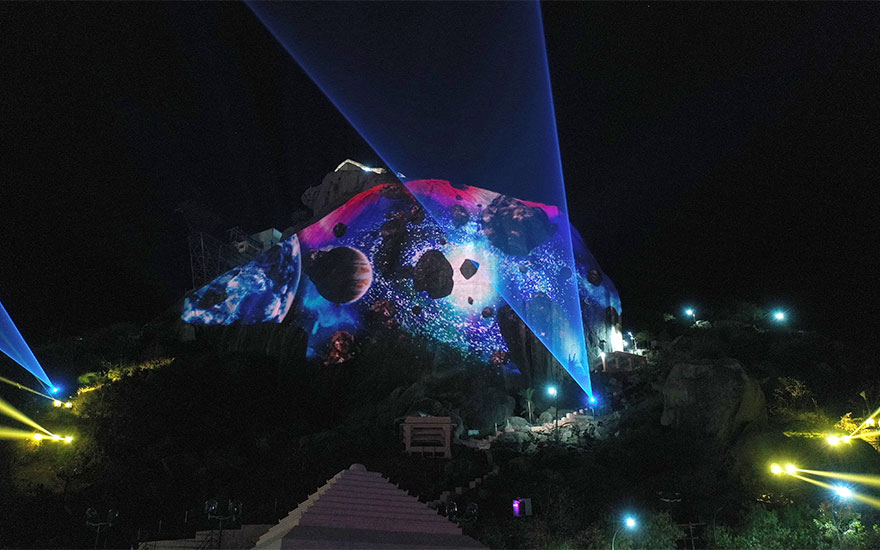A horizontally oriented, nighttime scene set against a black background showcases a blend of elements that make it challenging to determine whether it is a realistic photograph, a computer-edited image, or a computer-animated graphic. The scene features a faint beige pyramid at the bottom, scattered with blue and yellow lights, some of which emit laser beams or triangular lights. 

In the dark foreground, there appears to be a poorly lit mountain-like structure. Central to the image, a swirling composition of red, blue, and white colors evokes the appearance of planets, asteroids, and perhaps a black hole or galaxy, adding to the celestial theme. A prominent planet resembling Jupiter is visible, along with many asteroids hovering on the horizon of a rocky planet, which has multiple searchlights that could be spaceships or robots.

A pagoda with a pyramid-shaped roof, set among what could be trees and other foliage, hints at terrestrial elements blending into the scene. Additionally, there are small blue lights emitting rays in a cone pattern toward the sky, possibly representing searchlights or some other form of illumination.

This intricate and imaginative depiction, potentially an artist's rendering or AI-generated image, lacks text but integrates various illogically ordered yet cohesive elements, creating an enigmatic and intriguing visual feast.